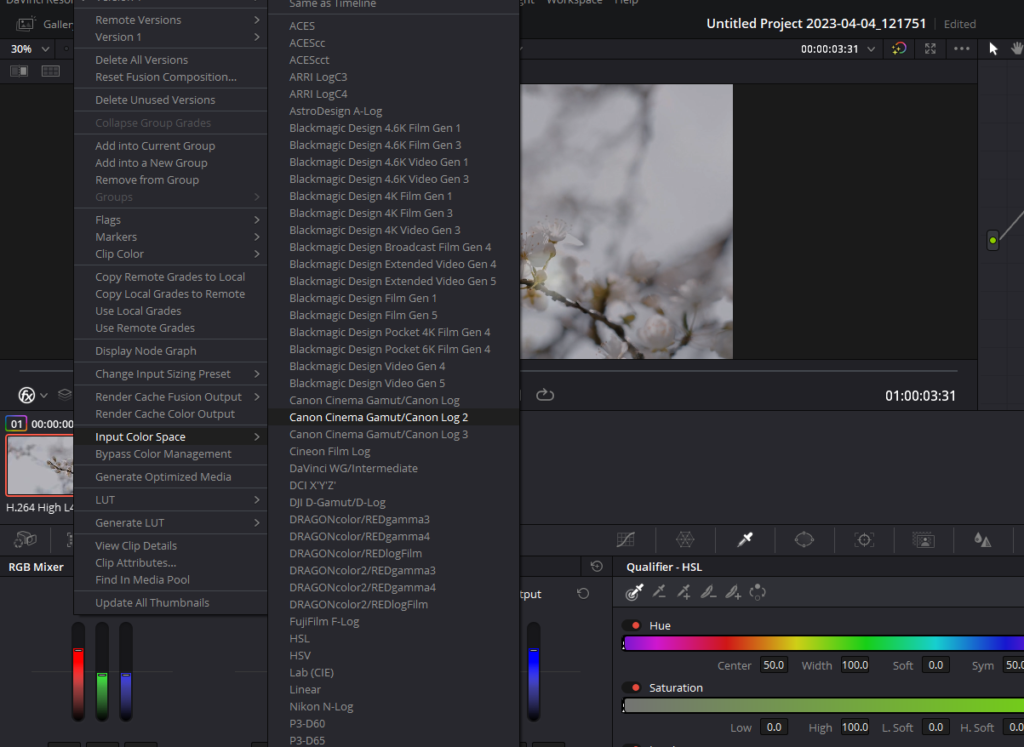This is a detailed screenshot of a video editing or color grading program, characterized by a predominantly dark gray user interface. The central focus of the display is a vibrant image of cherry blossoms, saturated with pink and white hues, against the gray backdrop. Situated above this image is a slightly lighter gray header, and beneath it, in the bottom-right corner of the footer, is the timestamp "01:00:03:31" in white text.

Two pop-up menus partially obscure the central still frame of the video, effectively covering about half of the image. The left pop-up menu contains a list of options, each segmented by thin light gray lines for better readability. The detailed contents of the left menu are as follows:

- **Remote Versions**
- **Version 1**
- **Align**
- **Delete All Versions**
- **Reset Fusion Composition…**
- **Align**
- **Delete Unused Versions**
- **Align**
- **Collapse Group Grades** (grayed out)
- **Align**
- **Add into Current Group**
- **Add into New Group**
- **Remove from Group**
- **Groups** (grayed out)
- **Align**
- **Flags**
- **Markers**
- **Clip Color**
- **Align**
- **Copy Remote Grades to Local**
- **Copy Local Grades to Remote**
- **Use Local Grades**
- **Use Remote Grades**
- **Align**
- **Display Node Graph**
- **Align**
- **Change Input Sizing Preset**
- **Align**
- **Render Cache Fusion Output**
- **Render Cache Color Output**
- **Align**
- **Input Color Space** (highlighted in dark gray)
- **Bypass Color Management**
- **Align**
- **Generate Optimized Media**
- **Align**
- **LUT**
- **Generate LUT**
- **View Clip Details**
- **Clip Attributes**
- **Find in Media Pool**
- **Update All Thumbnails**

The right pop-up menu, which lacks the segementing lines of the left menu, contains multiple lines of text, continuing the interface's cohesive and detailed layout. These elements combine to form a comprehensive and user-centric interface for the video editing or color grading software, crucial for professionals aiming for precise and refined control over their visual projects.